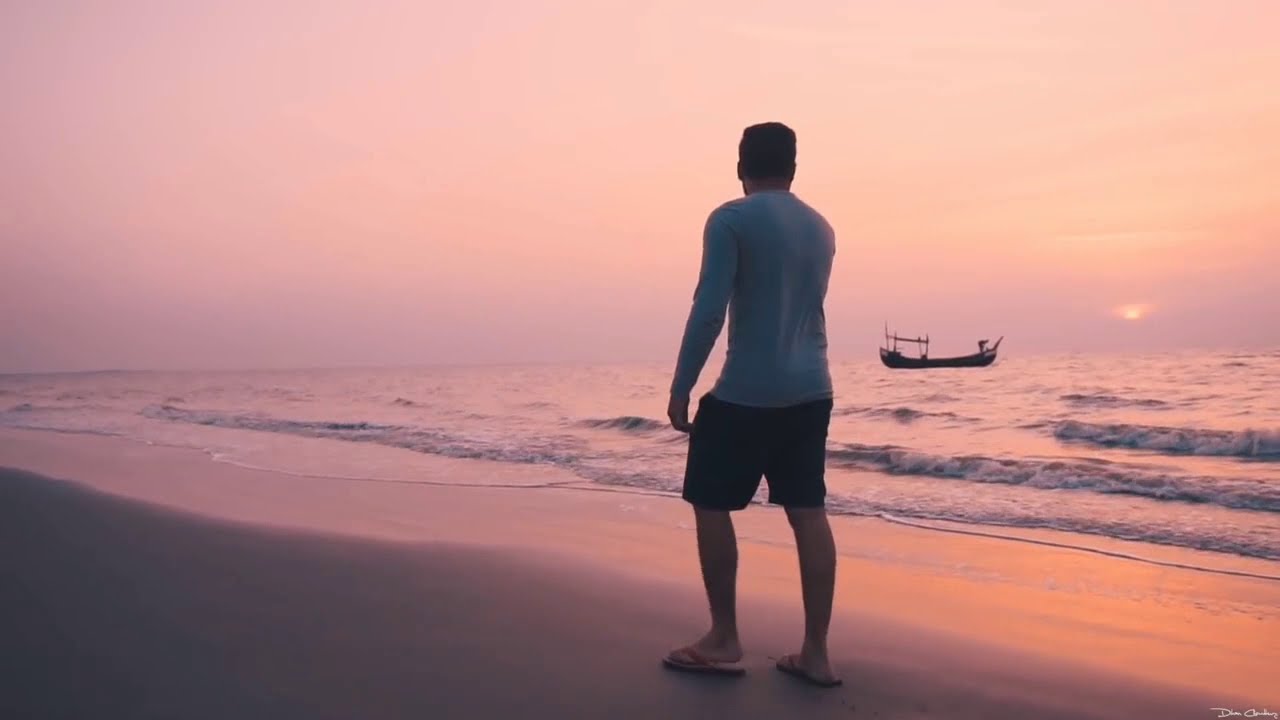The photograph captures a serene beach scene during what appears to be either sunrise or sunset, characterized by an overcast sky tinged with pink and peach hues. A muscular, Caucasian man with brown hair stands at the edge of the beach, facing away from the camera. He is dressed in a form-fitting, long-sleeved white shirt, dark shorts, and flip-flops. The wet sand beneath him is smooth and undisturbed, reflecting the soft golden glow of the sun as it peeks through the clouds. Gentle waves lap at the shore in front of him, indicating shallow waters. In the distance, a shadowy silhouette of a small fishing boat can be seen near the horizon, contributing to the tranquil ambiance of the scene.